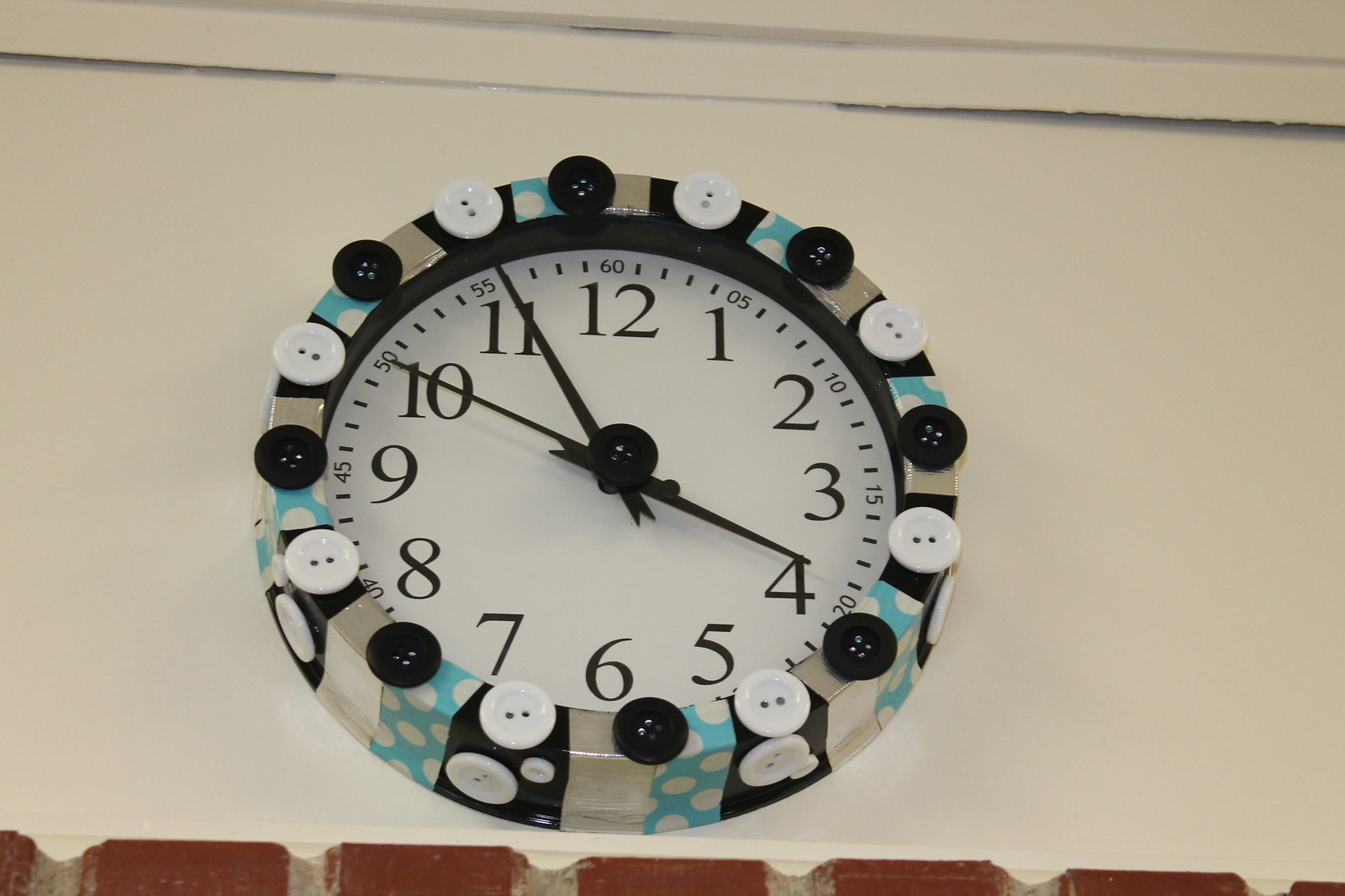The image depicts a high angle view of a white wall, with a ceiling in the top right corner and a section of red bricks at the bottom. The focal point of the photograph is a round clock mounted on the wall. The clock is uniquely decorated with alternating strips of blue with white polka dots, shiny off-white, and black materials around its outer edge, giving it a crafted appearance. The clock frame is further embellished with black and white buttons. The clock face is white, displaying bold black numbers from 1 to 12 and minute indicators at five-minute intervals from 05 to 60. The clock has three black hands indicating the hours, minutes, and seconds. The time shown on the clock is approximately five minutes to four.